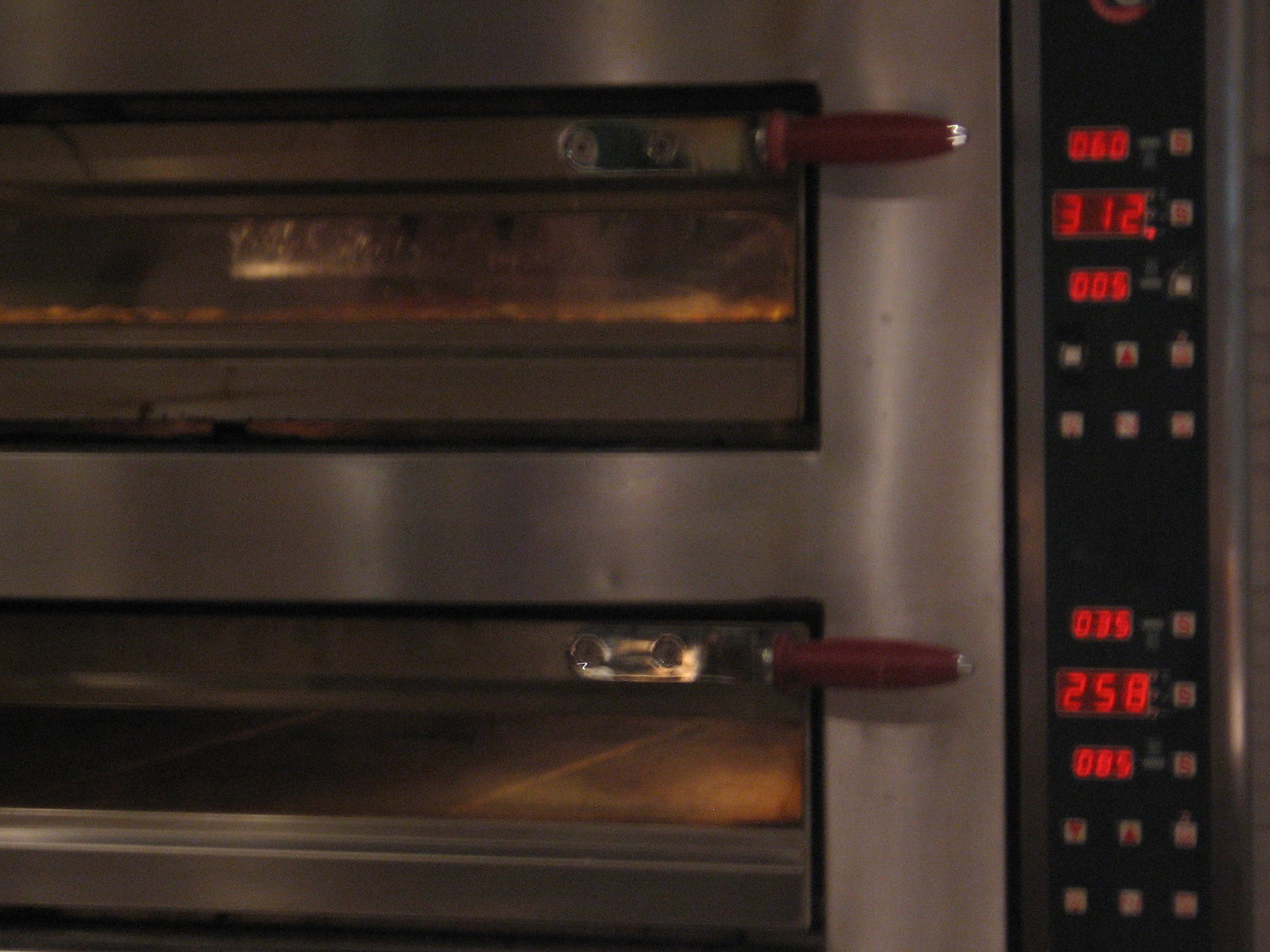This image showcases a commercial-grade, stainless steel double oven, likely designed for industrial or restaurant use, with distinct features indicating it is potentially a pizza oven. The ovens are stacked with one on top of the other, both featuring burgundy wooden handles for opening their respective doors which are equipped with glass windows for viewing the interior. The control panel, located on the far right-hand side, displays digital red numbers indicating various settings and times: the top oven reads "060," "312," and "005," while the bottom oven displays "035," "258," and "085." Both ovens have three rows of indicator lights and six buttons for operating different functions. The image appears to be zoomed in, and the top oven has something cooking inside, possibly pizza or flat food items, while the bottom oven remains empty. The overall equipment is partially cut off on the left-hand side, but its industrial size and detailed control panel suggest it is a high-capacity appliance suitable for commercial kitchens.